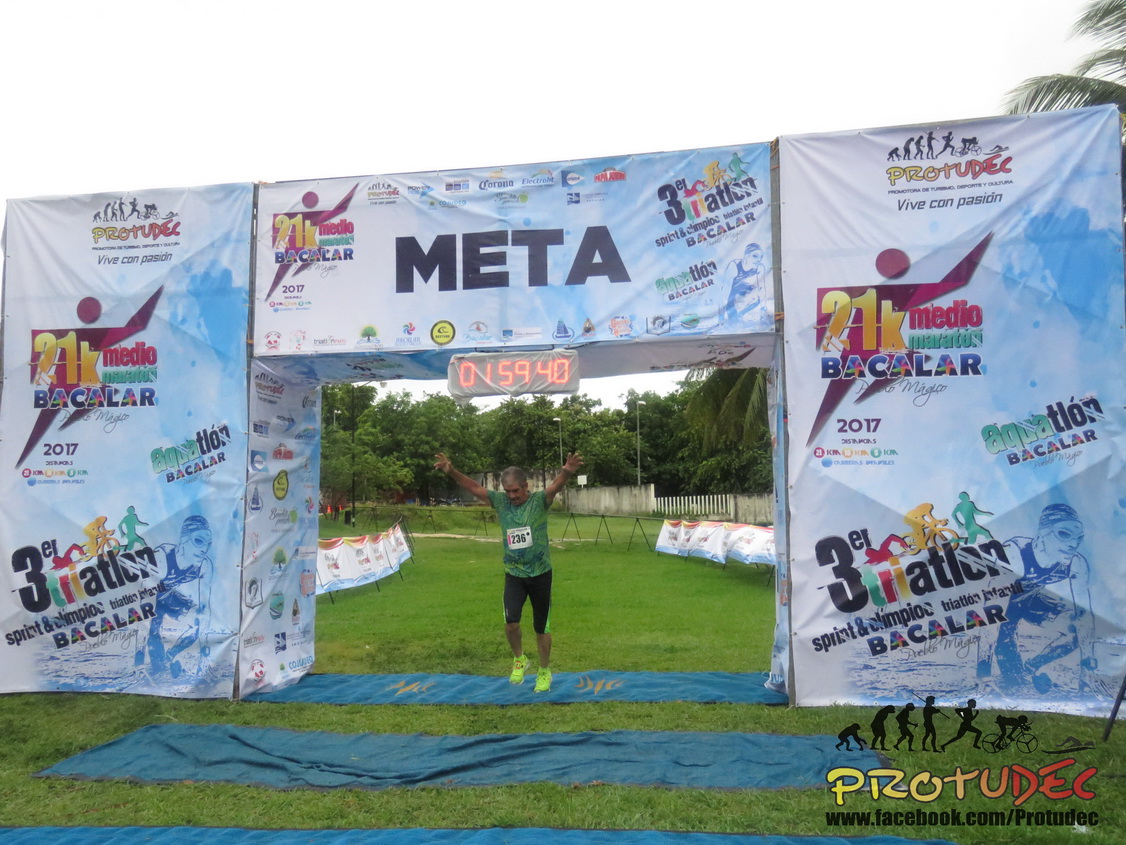In this vibrant photograph, an older Hispanic man is captured celebrating his finish at a race, having crossed the finish line with his hands triumphantly raised in the air. He is dressed in running gear: a green and blue short-sleeved shirt with a runner’s number, 236, emblazoned in a white square on the front, black knee-length spandex pants, and bright yellow running shoes. He stands on a blue carpet that stretches across a large grassy area, with multiple barricades also adorned with signs and logos in the background.

Above him looms an arch-like finish line structure comprising two pillars and a horizontal banner, both covered in various logos and text. The most prominent logo, in bold black letters, reads "META," which is centered on the banner. Other logos on the pillars include "21K Makato Marathon," "Barclay," "Meteo," "Bacolar," and more, indicating a possible international event. Below the banner, a large black timer clock displays the race time: 01:59:40 with bright red digits. Intriguingly, the lower right corner of the image features additional text and illustrations, including an evolutionary diagram and the words "Pro2 Dec" (P-R-O-T-U-D-E-C), alongside a link to www.facebook.com/P-R-O-T-U-D-E-C.

Overall, this image powerfully captures the climactic moment of the runner's achievement, set against the backdrop of a well-organized and celebratory race finish line.